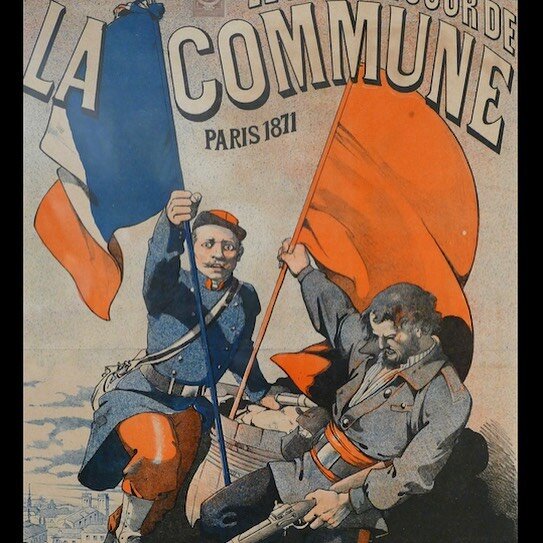The image is an old magazine cover or poster, likely originating from 1871, judging by the dated style and attire. The background is a light gray, and at the top, bold white block letters spell out "La Commune" with "Paris 1871" printed below in smaller text. The central illustration depicts two soldiers. The soldier on the left is dressed in a blue uniform with red pants and a red cap; he carries a blue flag with blue, white, and red stripes, reminiscent of the French flag. He also appears to have a sling over his shoulder, possibly for a canteen, and is standing near a barrel. The soldier on the right, slouched and seemingly wounded or dead, has a head injury marked by a hint of red. He wears a gray jacket with an orange cummerbund and holds a downward-pointing gun in his left hand, while also gripping a solid orange flag. The bottom left corner of the illustration shows buildings, adding to the setting's authenticity by suggesting a Parisian backdrop. The scene evokes a realistic depiction of wartime, contributing to the historical narrative suggested by the title and date.